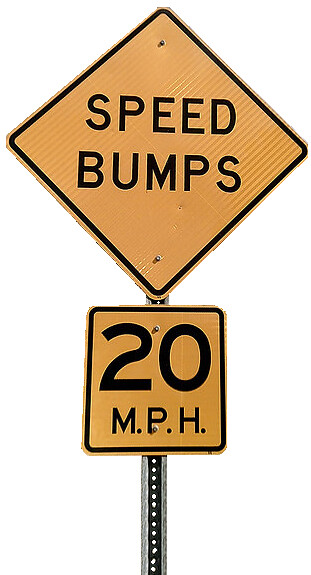The image depicts a traffic control sign set against a white background. The sign is mounted on a gray steel pole that features evenly spaced holes along its length. The pole is secured with bolts, and we see portions of it, including where the signs are attached.

At the top, there's a diamond-shaped, yellow warning sign with a black trim. In bold, black, capital letters, it reads "SPEED BUMPS." Below this, attached to the same pole, is a square, yellow sign with similar black trimming. This sign displays a speed limit of "20 M.P.H." in black digits and letters. The signs are fastened to the pole by visible screws or bolts – four in total, positioned at the top and bottom points of the diamond sign and at the top and midpoint of the square sign. There are no other signs or attachments visible on the pole.

The overall presentation highlights the cautionary message of the signs, their sturdy mounting, and the minimalist yet clear design against the white backdrop.